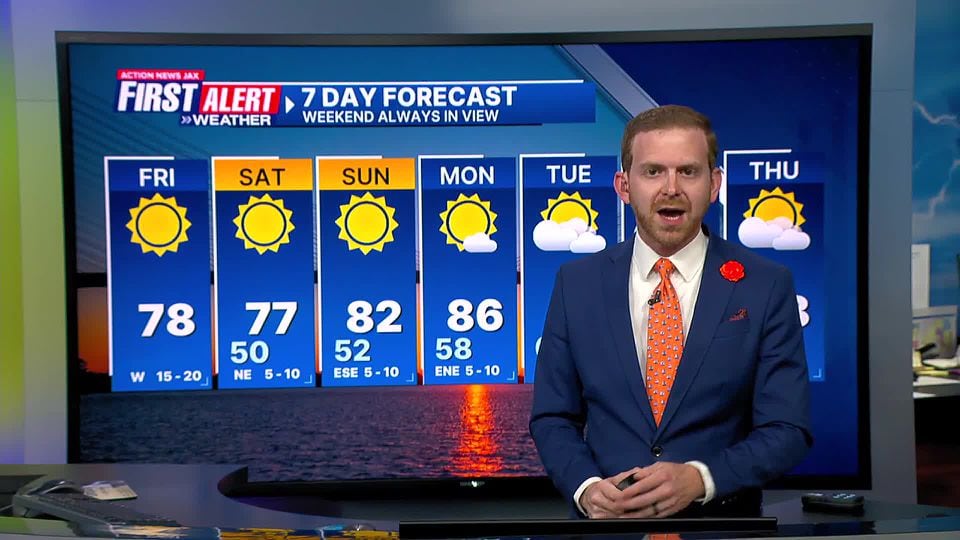This still image from an evening news weather segment features a Caucasian weatherman standing confidently before a large video monitor and a semi-circular brown wood desk. He is dressed in a sharp navy blue three-piece suit, complemented by a white button-down shirt, an orange patterned tie, and a matching orange flower pinned to his lapel. He stands with his hands clasping a remote, facing slightly to the right of the screen. Behind him, the large video monitor prominently displays the "First Alert Weather: Seven Day Forecast" with the tagline "Weekend Always in View," along with the daily forecasts from Friday through Thursday. The background of the screen showcases an ocean view with a picturesque setting sun, adding a serene touch to the informative weather segment. Portions of the news studio wall and workspace are also visible beyond the monitor. The forecast predicts sunny conditions transitioning to cloudy skies with temperatures ranging from 77°F to 86°F.